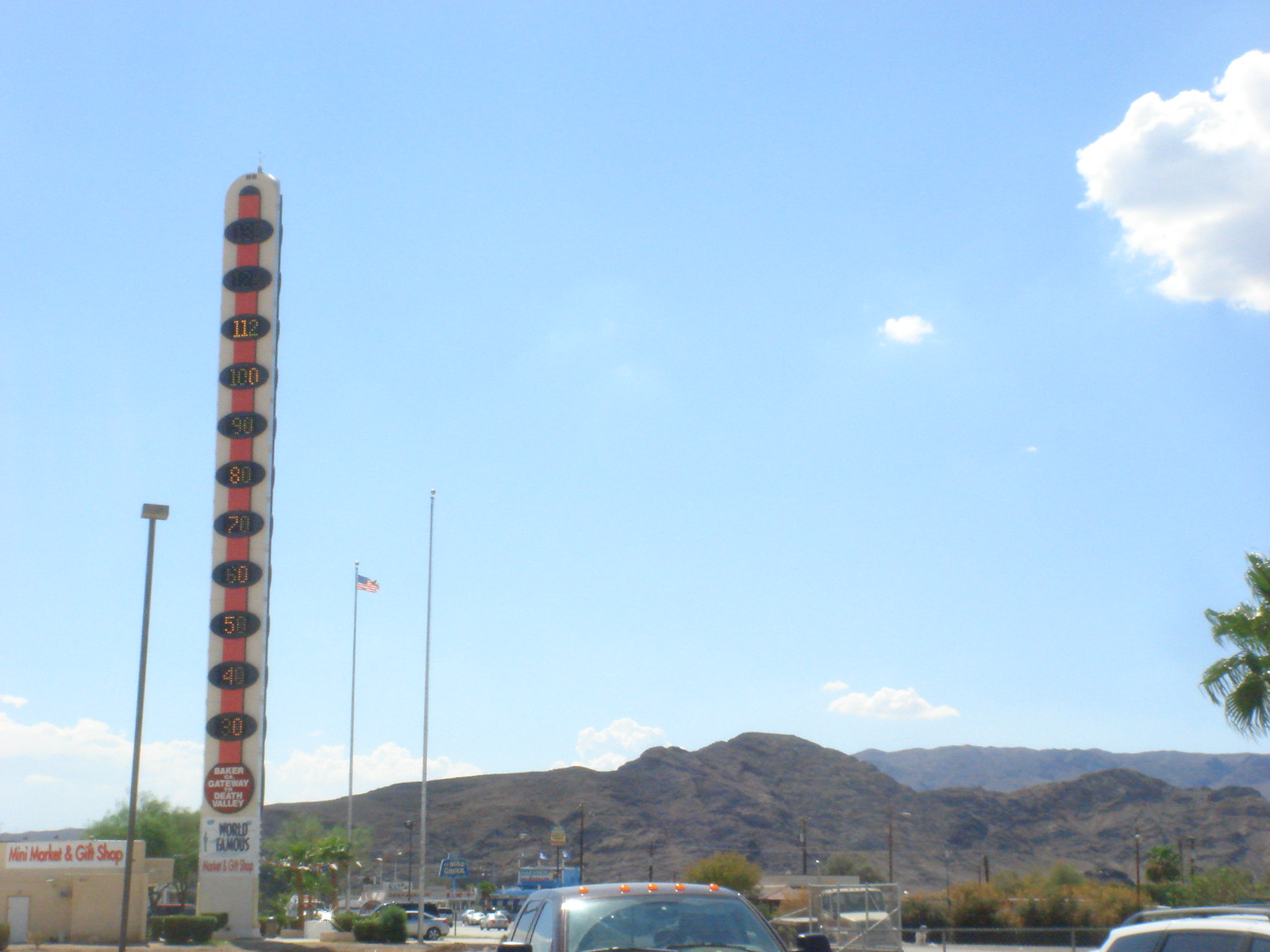This photo captures a parking lot set against a backdrop of a clear, vivid blue sky. The image is taken from a distance, making the finer details less discernible. Dominating the scene is an elevated structure with an orange bar that stretches above the parking lot, interspersed with evenly spaced black ovals. Each oval appears to have numbers on it, though they are not clearly readable. Several light poles dot the parking lot underneath this structure. In the far background, arid, desert-like mountains rise up, adding a rugged contrast to the otherwise structured setting. Soft, scattered white clouds drift across the sky, enhancing the photo's depth and tranquility.